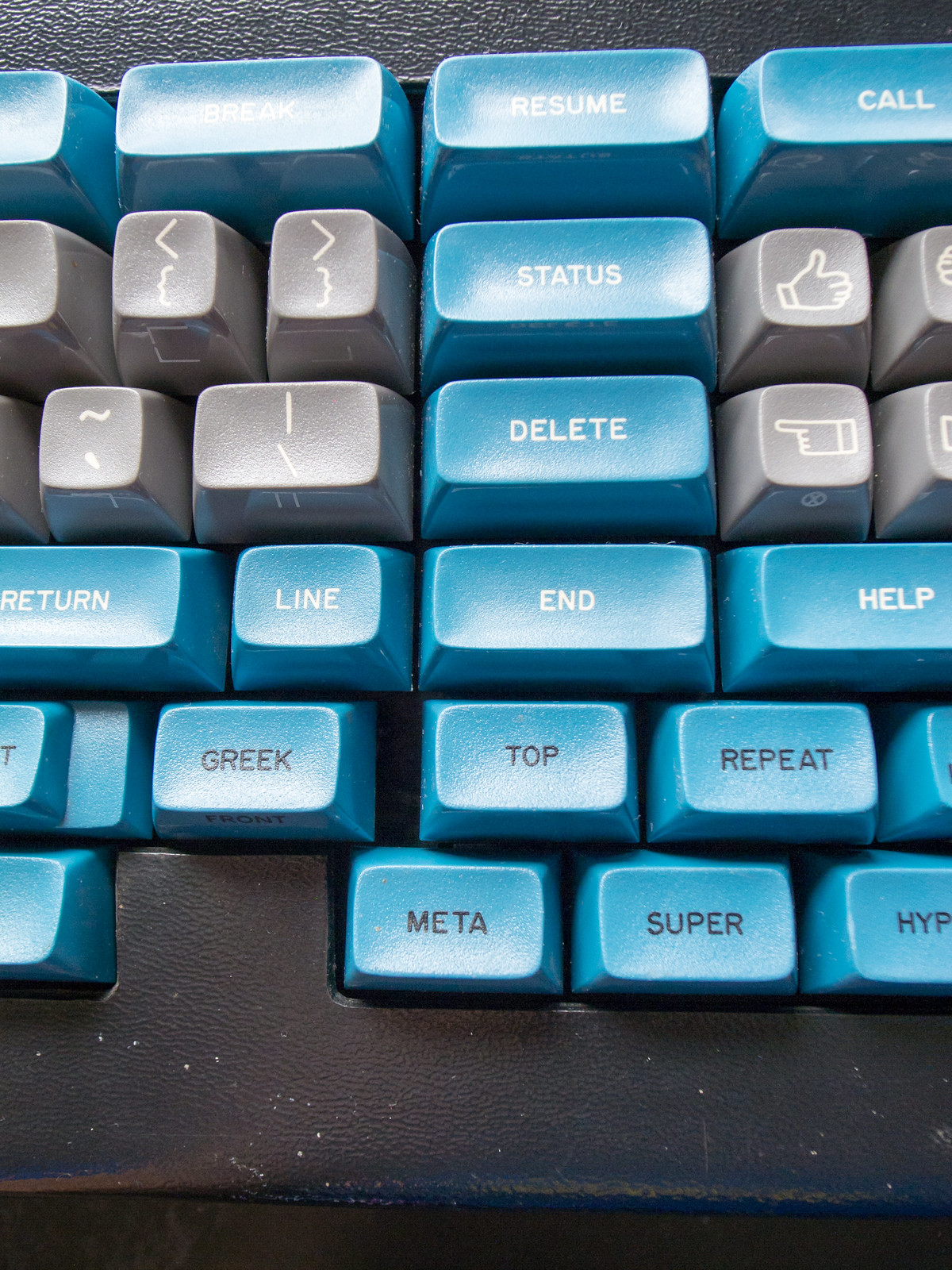This photograph, oriented in portrait, captures the center of an unusual and specialized keyboard set against a black frame. The keycaps are primarily gray and vivid blue, and they feature various functions written in contrasting white or black text. At the top, large blue keys prominently display words such as Resume, Call, Status, Delete, Return, Line, End, and Help. Below these, additional blue keys list Greek, Top, Repeat, Meta, and Super. The gray keys are adorned with a variety of symbols, including a left-pointing thumbs up, less than and greater than signs, a slash, a tilde, and others. Overall, this striking keyboard section hints at a unique and specialized purpose, differing significantly from a typical keyboard.